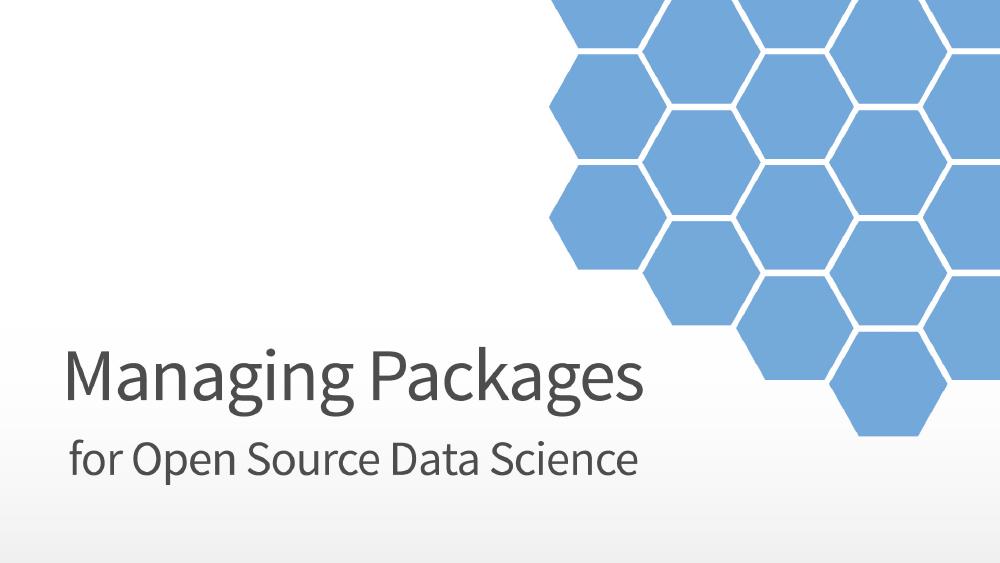An image showcases what appears to be a title or cover page for a presentation. The background is entirely white, with a light blue honeycomb pattern extending from the lower right corner and gradually fading as it moves towards the center. Prominently displayed at the top in large letters are the words "Managing Packages," while just below in a smaller font it reads "For Open Source Data Science." This clean and modern design hints at a professional and organized topic likely focusing on data management within the field of open-source scientific computing.